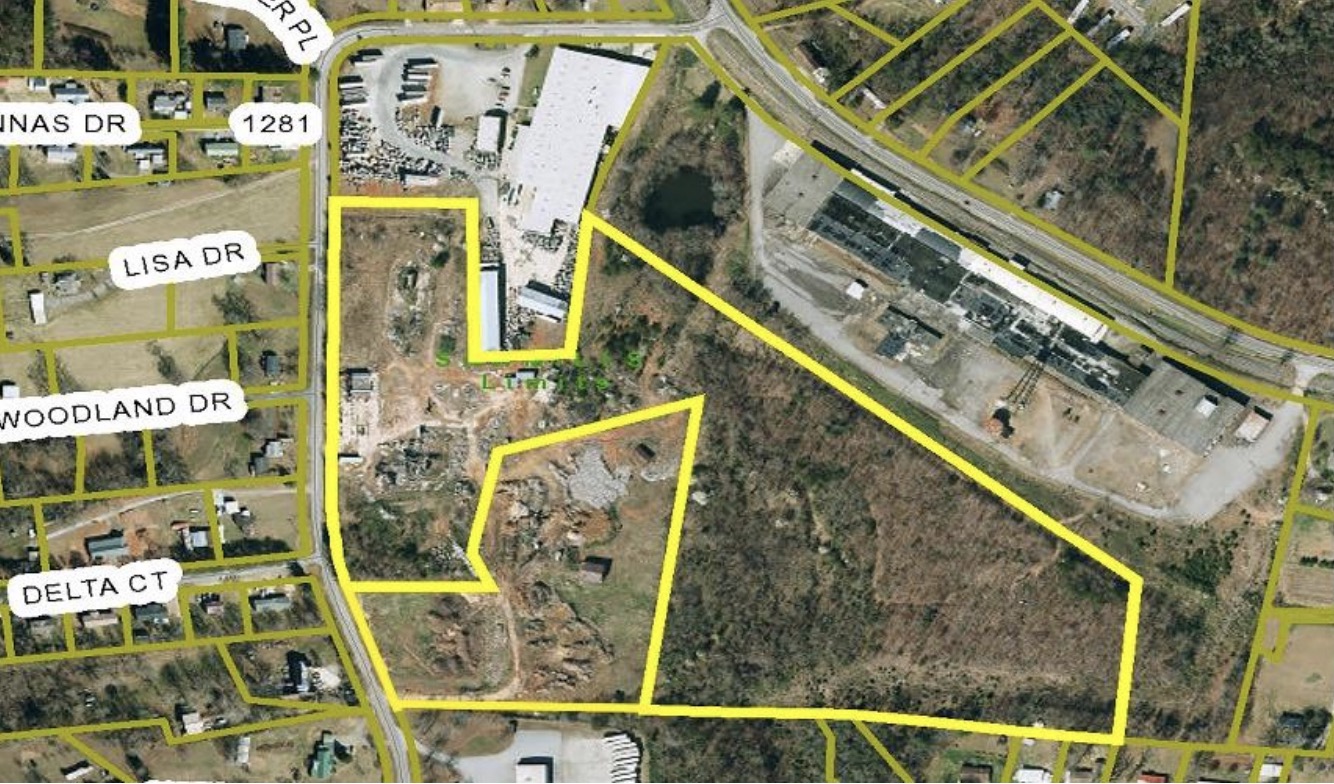The image is an aerial map resembling a Google Maps view, showcasing a mixed residential and commercial neighborhood. The map prominently features yellow lines outlining different land parcels, likely indicating ownership boundaries or construction sites. The left side of the image includes street names such as Lisa Drive, Woodland Drive, and Delta Court, marked with white labels and black letters. In the topography, you can discern sections of grass, wooded areas, and a few houses represented by small squares. The right side of the image appears to be dominated by commercial properties or potential businesses, possibly hinting at a shopping mall. The color palette includes greens, browns, grays, whites, and blacks, providing a typical bird's-eye view with little detail on individual buildings. The streets are highlighted in thick olive-colored lines, weaving through the area, giving a well-defined layout of this town.